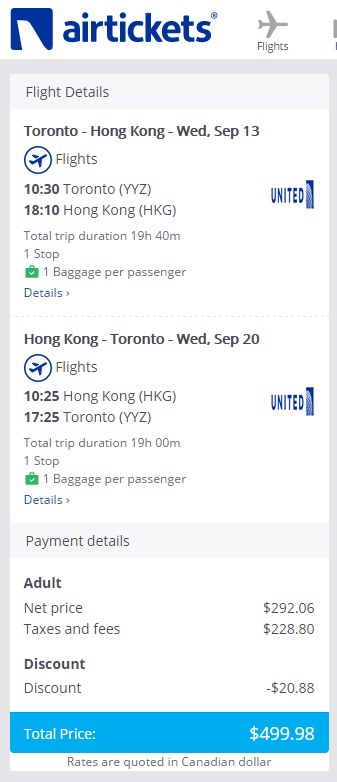**App Screenshot: AirTickets - Toronto to Hong Kong Flight Details**

At the top of the screenshot is the app name "airtickets" written in blue lowercase letters, accompanied by its blue and white logo featuring the fin of an airplane. On the right-hand side, the word "Flights" appears next to an airplane icon. 

Below this header, a gray bar contains the label "Flight Details." The main section below lists the search results within white boxes.

**Flight Information: Toronto to Hong Kong**
- **Date:** Wednesday, September 13
- **Flight:** 
  - Departure: 10:30 AM from Toronto (YYZ)
  - Arrival: 6:10 PM in Hong Kong (HKG)
- **Total Trip Duration:** 19 hours and 40 minutes
- **Stops:** One
- **Baggage:** One checked bag per passenger
- **Details:** Option to view more information with an arrow button
- **Airline:** United Airlines (logo displayed)

**Return Flight: Hong Kong to Toronto**
- **Date:** Wednesday, September 20
- **Flight:** 
  - Departure: 10:25 AM from Hong Kong (HKG)
  - Arrival: 5:25 PM in Toronto (YYZ)
- **Total Trip Duration:** 19 hours
- **Stops:** One
- **Baggage:** One checked bag per passenger
- **Details:** Option to view more information with an arrow button
- **Airline:** United Airlines (logo displayed)

**Payment Details:**
- **Adult Net Price:** $292.06